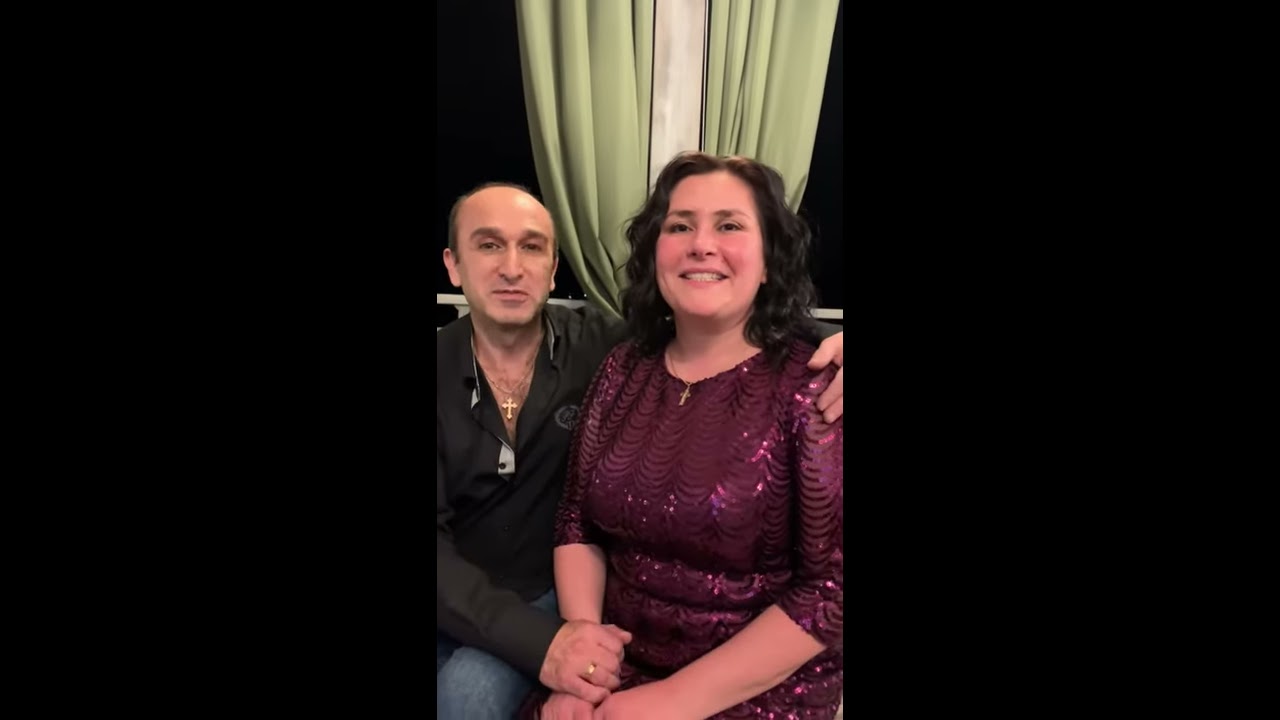The image features a couple sitting closely together, presented in a central frame with black sections on either side. The woman, who has wavy brown hair and dark brown eyebrows, is dressed in a burgundy sequin dress with sleeves that reach just past her elbows. She sits with a radiant smile, revealing her teeth, her hands gently crossed on her lap. Around her neck, she wears a cross necklace. The man beside her, slightly older with thinning hair on top, is dressed in blue jeans and a long-sleeved black button-up shirt with a few buttons undone. He also sports a gold cross necklace and a gold wedding band on his hand, which rests tenderly on the woman's hands. They are both looking directly at the camera. The background suggests they are on a patio, emphasized by a white metal railing and tied-up green and white curtains illuminated by natural light.